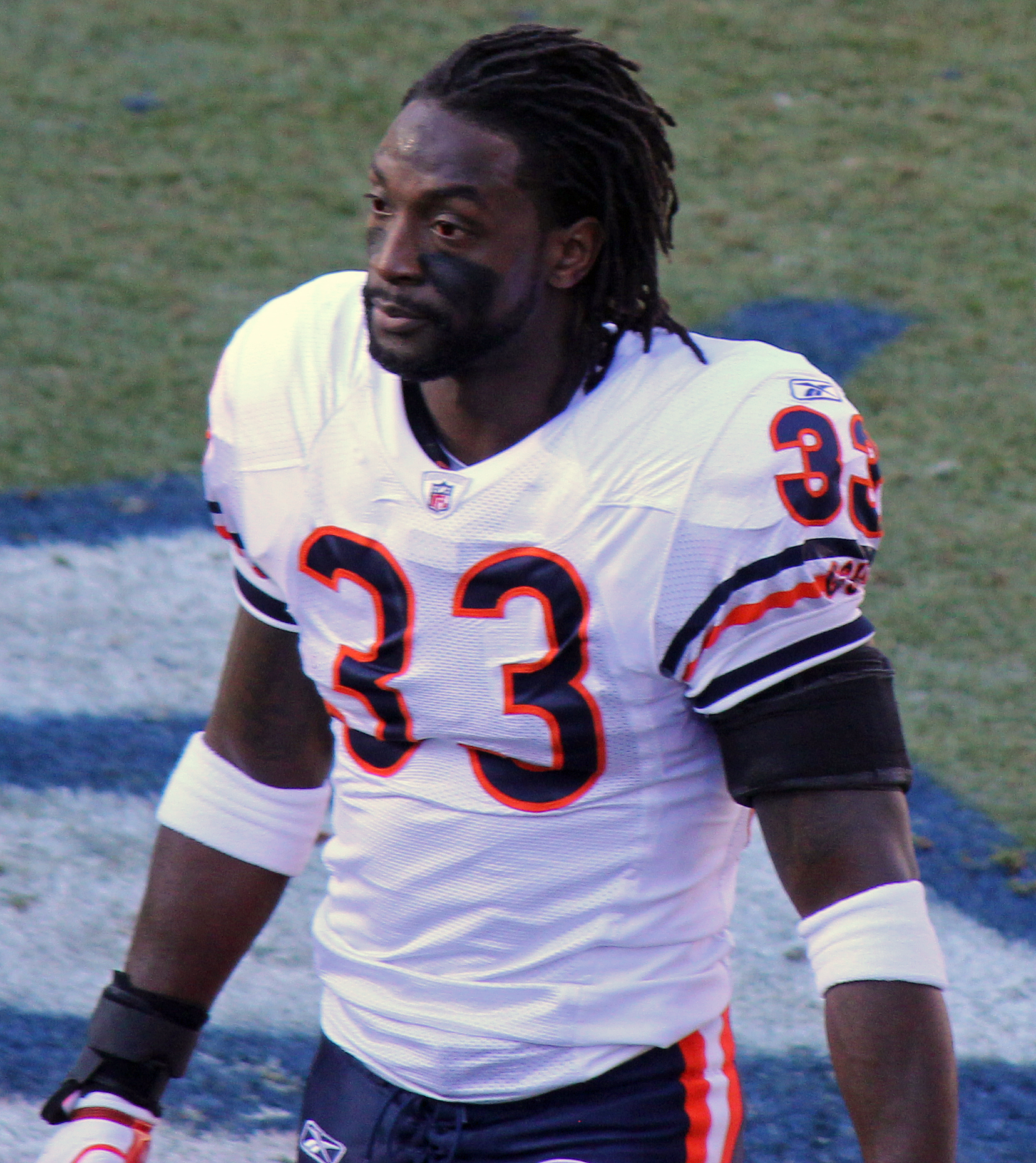This detailed color photograph captures an American football player in the middle of a game. He stands prominently at the center of the image, set against a backdrop of green grass with a partially visible blue and white logo, suggesting a football field. The player has black braided hair, black eye black under his eyes, and a goatee. He gazes off to the left, donned in a white NFL jersey featuring the number 33 in black, outlined in orange. His attire includes white wristbands near his elbows, white gloves on his right hand, and black pants adorned with orange and white stripes. The scene is alive with the vibrant colors of the field and the player's uniform, depicting the intense, focused atmosphere of a football game.